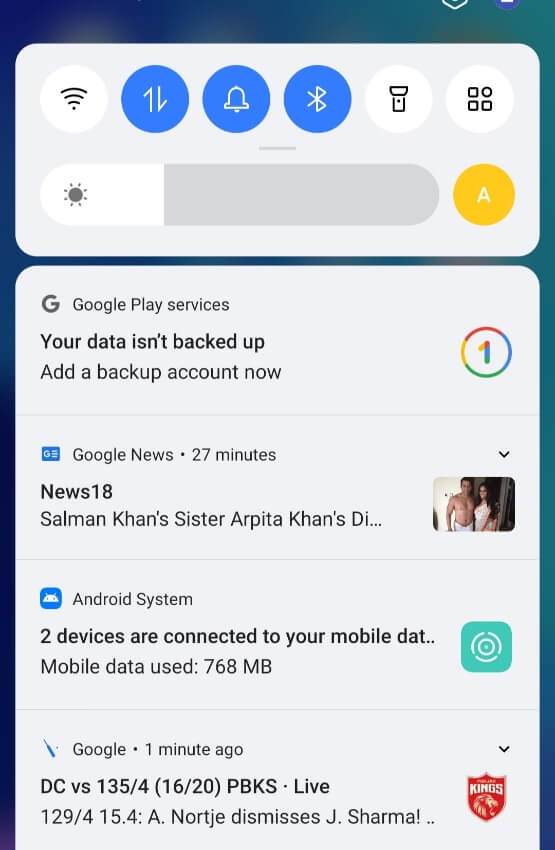**Detailed Caption:**

"This screenshot captures the settings page of a Samsung Galaxy smartphone, immediately identifiable by its distinct icons and layout. The status bar at the top of the screen displays the Wi-Fi strength indicator, the Bluetooth symbol, and notification alerts, confirming that Bluetooth is active. The flashlight and several other applications are also visible. Towards the middle of the screen, there's a setting for adjusting the screen brightness, currently set at approximately 30%. The text size appears to be adjusted as well.

Notably, various notifications populate the screen. One alert indicates that 'your data isn't backed up,' with an option to 'add backup account now.' Another notification mentions a Google News update from 27 minutes ago, reporting 'Salman Khan's sister are P2Cons,' with the rest of the headline truncated. Additionally, there's an important alert from the Android system stating, 'Two devices are connected to your mobile data,' with 768 megabytes of data having been used. Another notification can be seen but its details are not fully visible in the screenshot."